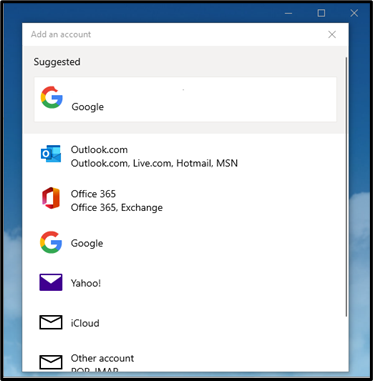Here is the cleaned-up and detailed caption:

---

A screenshot captured on a smartphone shows an email account selection menu. Dominating the screen's center is a white interface framed against a blue sky background, gradually transitioning to clouds towards the lower portion. At the top right corner, standard window controls are visible, including minimize, maximize, and close buttons.

The menu lists multiple email services, each paired with its logo:
1. **Google** with the multicolored 'G' logo.
2. **Outlook** featuring a blue 'O' inside a box. The associated domains listed are outlook.com, live.com, hotmail.com, and msn.com.
3. **Office 365** illustrated by a three-dimensional red box, tilted to one side.
4. **Google** again with the same multicolored 'G' icon.
5. **Yahoo** represented by an envelope icon.
6. **iCloud** also marked with an envelope icon.
7. **Other Account** partially visible at the very bottom, indicated by an envelope icon.

The clear layout and distinctive icons make this screenshot an informative guide for selecting different email account types on a mobile device.

---